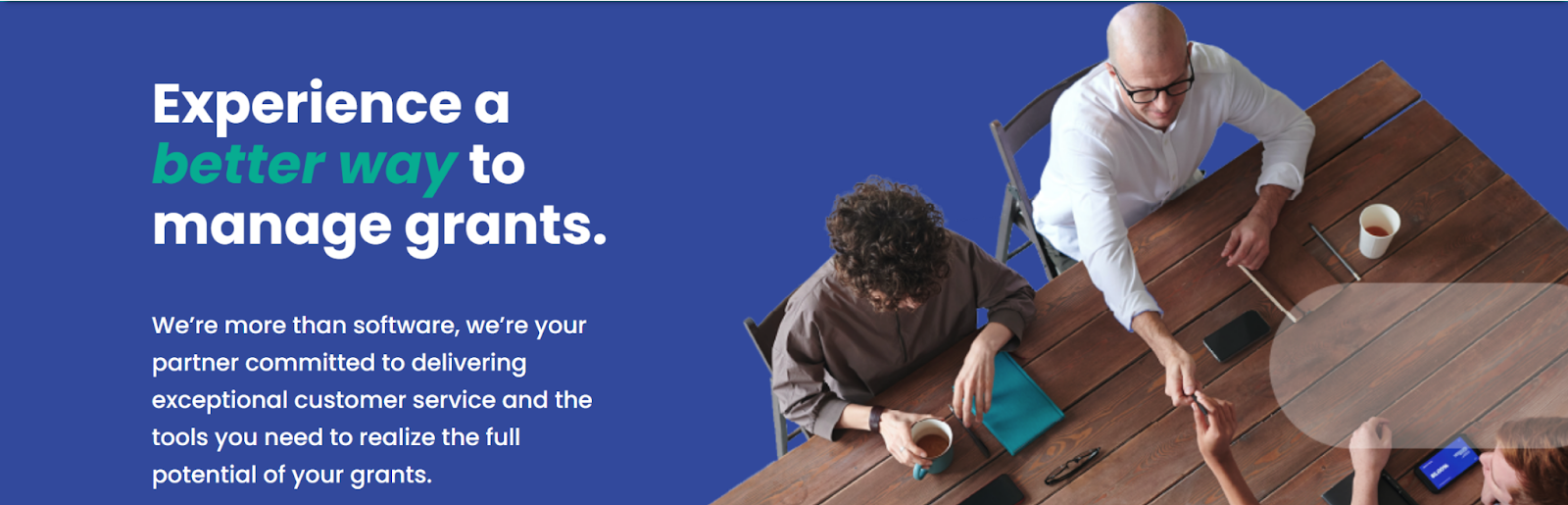A digital banner with a dark periwinkle background prominently features a captivating message to the left: "Experience a better way to manage grants," written in large letters. Notably, "better way" is highlighted in green, while the rest of the text is in white. Beneath this headline, smaller white text elaborates further: "We're more than software. We're your partner committed to delivering exceptional customer service and the tools you need to realize the full potential of your grants."

To the right side of the text, the image portrays two individuals seated at a table. The woman on the left is partially visible, holding a cup of coffee in her right hand and resting her left hand on a teal-colored book. Only the top of her head is shown. To her right sits a bald man with glasses, dressed in a white shirt. He appears to be handing something to someone across the table. In front of him, the table is adorned with a cup of coffee, a phone, and a pencil.